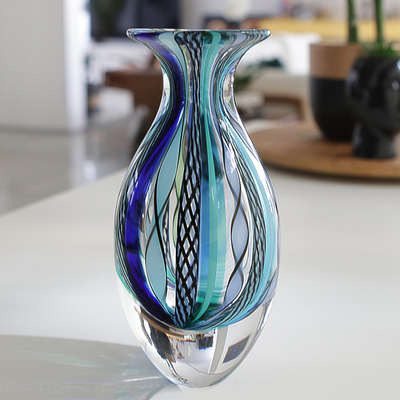This is a detailed photograph of an intricately designed glass vase resting on a white table. The vase, characterized by its shimmering, translucent surface, features an elegant curvaceous shape that bends inward at the upper third before flaring outwards towards its fluted top and bulbous bottom. Primarily clear, the vase is adorned with vertical linear designs in shades of blue, pale blue, turquoise, and green, enhanced with dark edges. These lines, resembling ribbons, twist and cross-hatch in a helix-like pattern, creating a visually captivating effect. The lower portion of the vase is notably thicker and more reflective, almost mirror-like, subtly warping the reflections around it. The table also holds a Lazy Susan and various small decorative items, while the softly blurred background hints at a cozy living room scene.